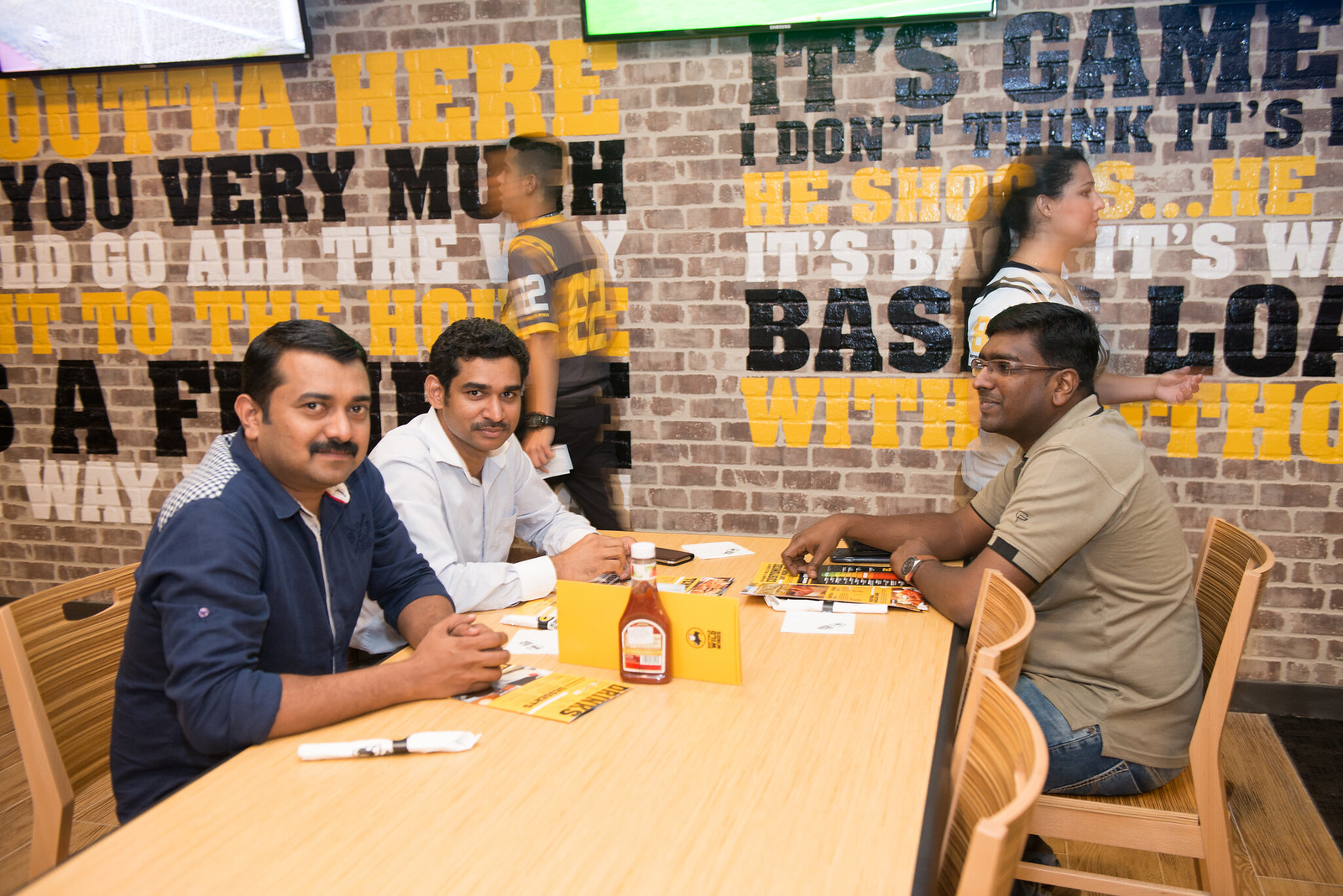The photo depicts three Indian men seated together at a wooden table in what appears to be a Buffalo Wild Wings restaurant, evidenced by the menus and the sports-themed phrases on the brown brick wall behind them. Two of the men, both sporting mustaches and wearing button-down shirts — one in beige and the other in light blue — are looking directly at the camera. Seated across from them is the third man with darker skin, engrossed in an open menu, dressed in a dark blue shirt with a watch on his left wrist. The table, which has no food yet, features three visible menus and a bottle of ketchup at its center. In the background, two blurred figures, a man and a woman, are walking in opposite directions, adding a dynamic element to the scene. The wall behind the men also includes painted text in yellow, black, and white, contributing to the lively atmosphere of the sports bar restaurant.